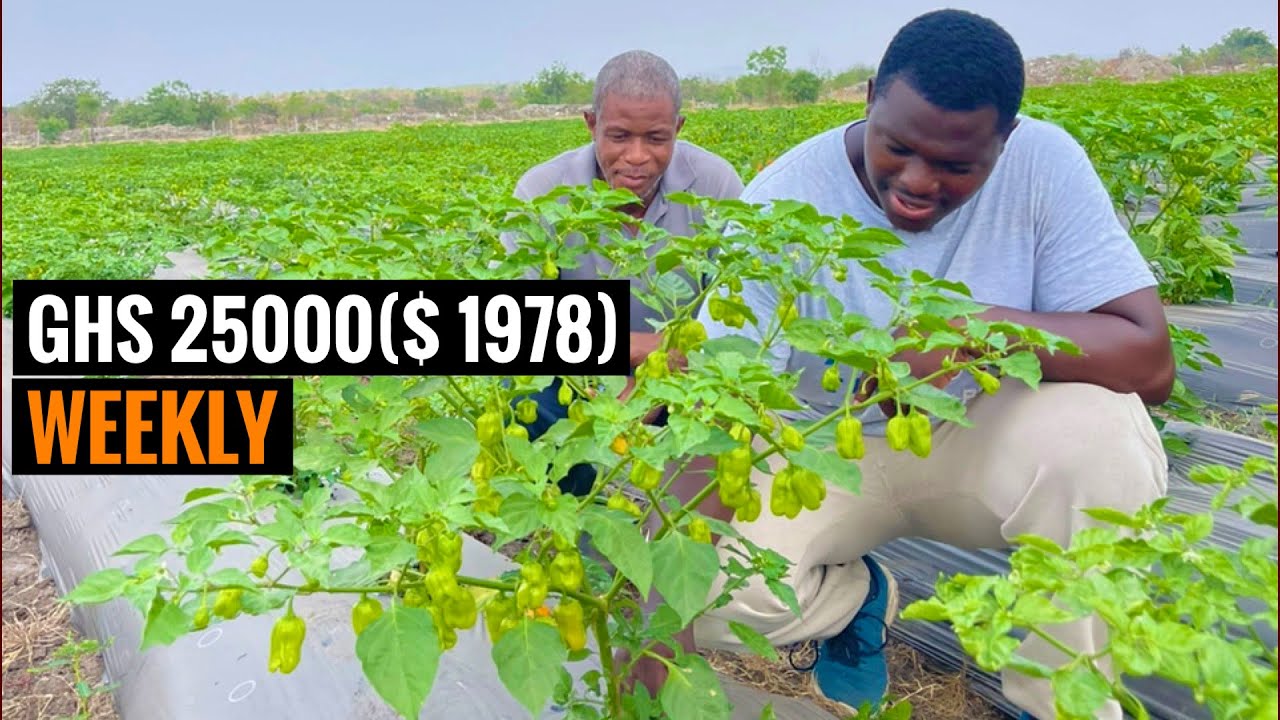This photograph, likely a YouTube thumbnail, was taken outdoors during a sunny day. It is rectangular, about 6 inches wide and 3 inches high, with a thin reddish-brown border framing the image. The central focus is a well-maintained field of crops, specifically rows of green bell pepper plants covered in gray plastic sheeting. The rows extend diagonally from the lower right to the upper left of the frame.

Crouched down near the center right of the image are two men of African descent, attentively examining one of the pepper plants, which feature tall, bushy vines with maturing green bell peppers that have hints of yellow and red. One man is wearing a blue t-shirt, white pants, and blue running shoes, while the other is dressed in a gray t-shirt and dark blue jeans. The background includes some taller trees and a clear periwinkle blue sky.

On the left side of the image, there are two black rectangles with text. The top rectangle contains white text that reads "GHS 25,000 ($1978)". The lower rectangle features orange text reading "Weekly". This suggests a monetary context, possibly related to earnings or profits from the cultivation of these peppers, which could be relevant to viewers familiar with Ghanaian currency. The overall composition and the strategically placed text give the impression of a staged, informative presentation, ideal for a YouTube thumbnail.